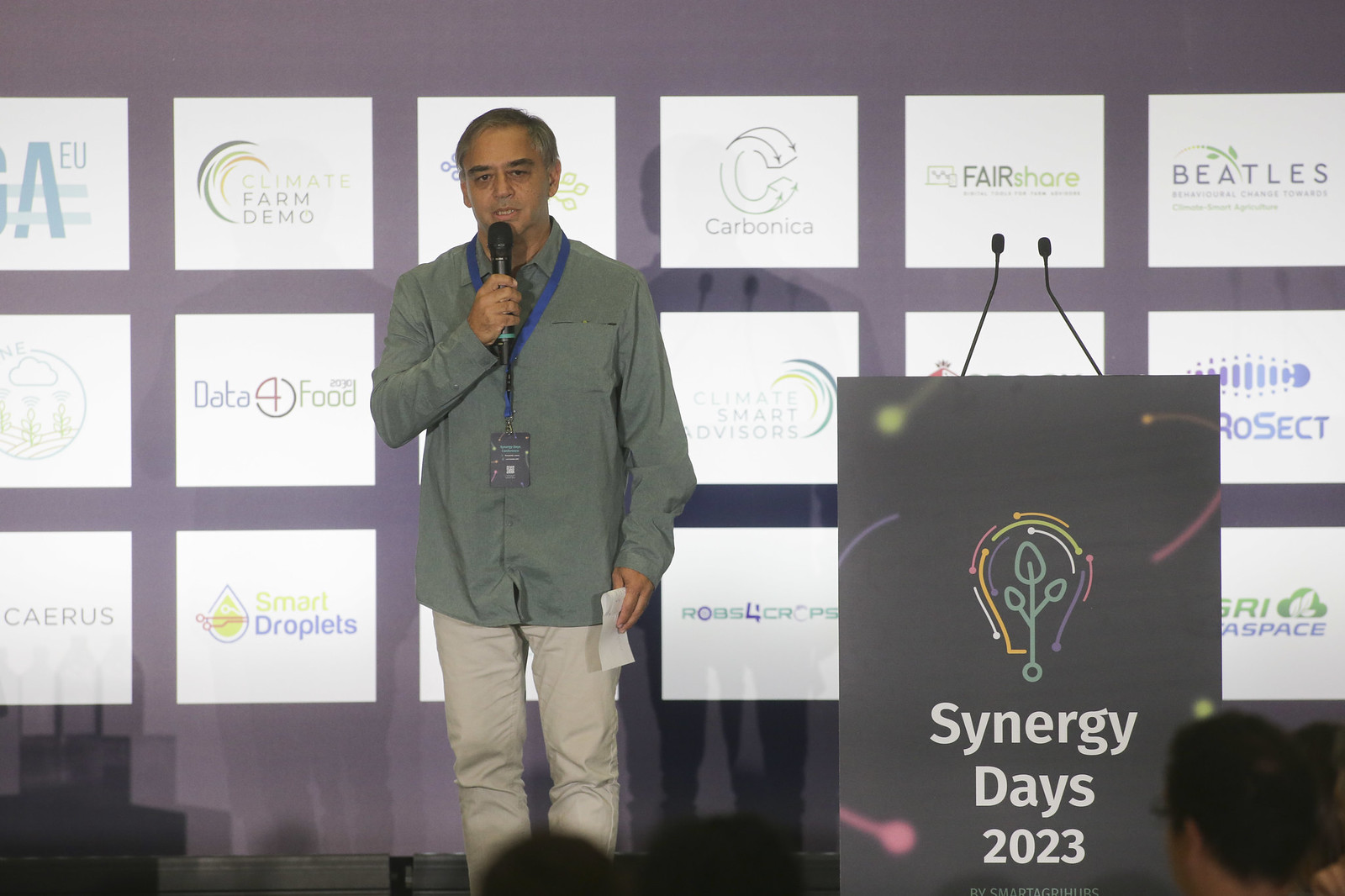The image portrays a well-groomed man with slightly dark skin and short brown hair with hints of gray, standing on a stage and addressing an audience. He is dressed in a neatly pressed long-sleeve button-down shirt, described variably as gray or green, untucked over casual khaki pants. Around his neck, he wears a blue lanyard with a badge. In his right hand, he holds a microphone close to his open mouth, clearly in the midst of speaking, while his left hand, resting by his side, holds a small piece of paper similar to the size of a receipt.

To the right of the man is a large podium adorned with a sign that reads "Synergy Days 2023," featuring a logo of a light bulb made up of different colored lines with a plant inside it. The podium sports two additional microphones, though the man stands apart from it. 

Behind him, a purple curtain serves as the backdrop, decorated with numerous rectangular white panels displaying various business logos and names, suggesting sponsorships or participants of the event. Some of the visible names include Climate Farm Demo, Data Food, Smart Droplets, Carbonica, Fair Share, and Beetles. 

In the foreground, the blurred backs of the audience's heads are faintly visible, emphasizing their focus on the man’s speech.